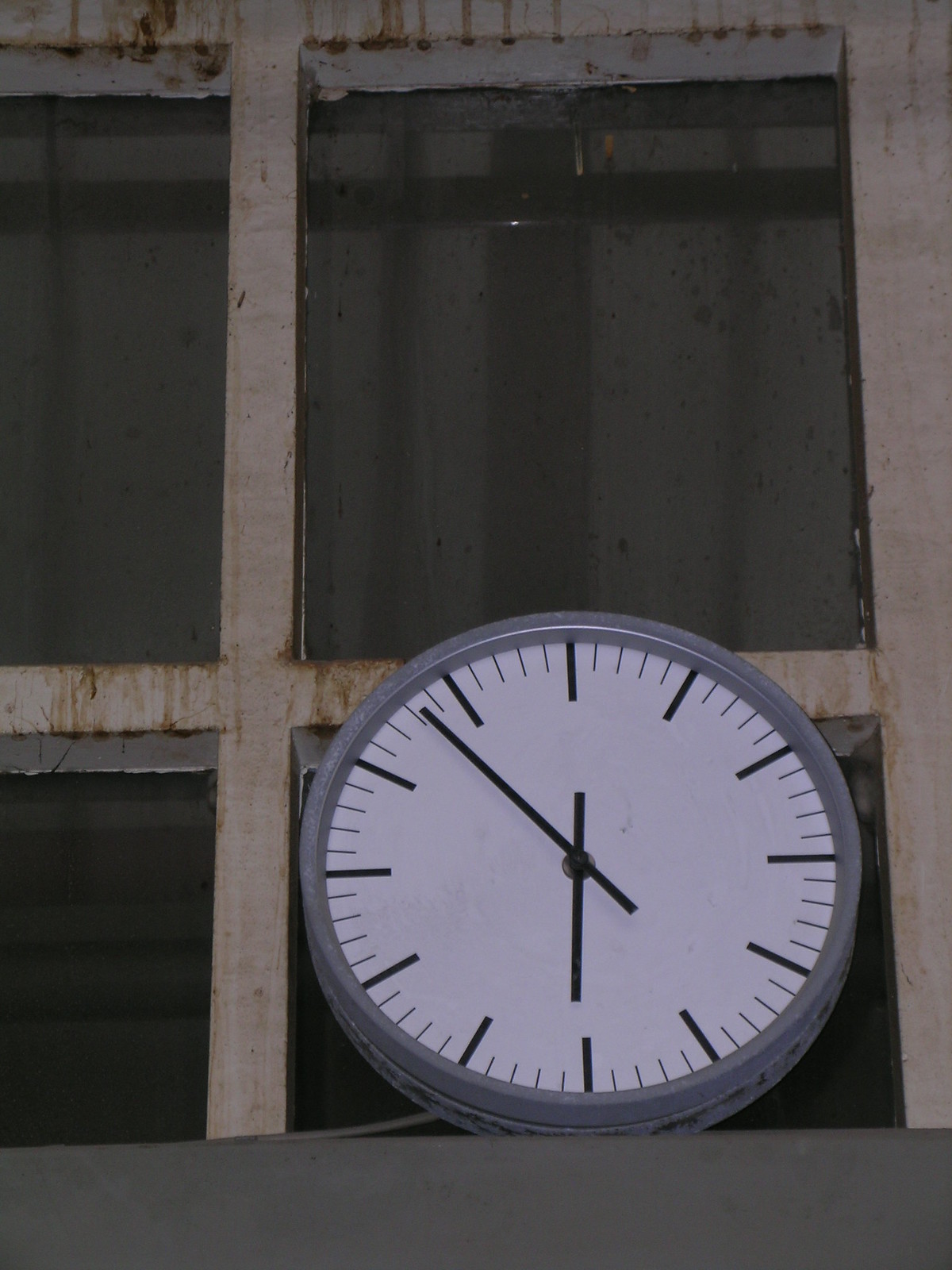This image captures an old, weathered window with a metal frame and dividers separating the panes of glass. The glass is notably stained and dirty, with streaks running down its surface, and the frame exhibits patches of rust indicative of age and exposure. A gray, round clock is mounted on the window, showing signs of wear with faded paint around its back ring. The clock features black minute and hour hands, but lacks numbers, instead displaying long thick black lines with four shorter, thinner lines in between each hour marker. Extending out from the back is a gray plug, contributing to the sense of disrepair and antiquity. The time on the clock appears incorrect, reading approximately seven minutes to seven.